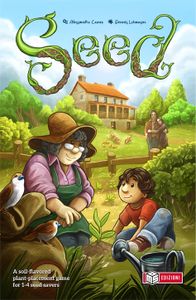This illustrated children's book cover, titled "SEED," exudes a serene gardening scene set against a backdrop of nature. The image is divided into distinct sections, with the top third showcasing a blue sky adorned with white clouds flanking each side. Dominating the center is the word "SEED," intricately crafted from green, sprouting plants. Below the title, a quaint brown house with an orange roof and a gray smokestack stands amidst lush greenery. The house features an orange front porch and is surrounded by vibrant trees and bushes.

A short brown wooden fence sits in front of the house, where two slightly out-of-focus figures embrace. In front, to the right, a small green bush adds to the verdant setting. By the bush, a little boy with shaggy brown hair, dressed in a red shirt, blue jeans, and brown shoes with white tips, sits on the ground. He has one leg over the other and is leaning forward, looking up to his left at an elderly woman. She wears a brown hat, glasses at the tip of her nose, a pink button-up shirt with rolled-up sleeves, and a green apron. The boy and the woman share a tender moment, focused on a small green plant with four leaves emerging from a dirt pile between them.

Additionally, a brown-and-white bird perches on a brown sack near the woman's shoulder, while another bird faces the duo from a green sack on the ground. Completing the picturesque scene, a watering can with its spout and handle visible sits next to the boy, emphasizing the gardening theme that ties the cover together.